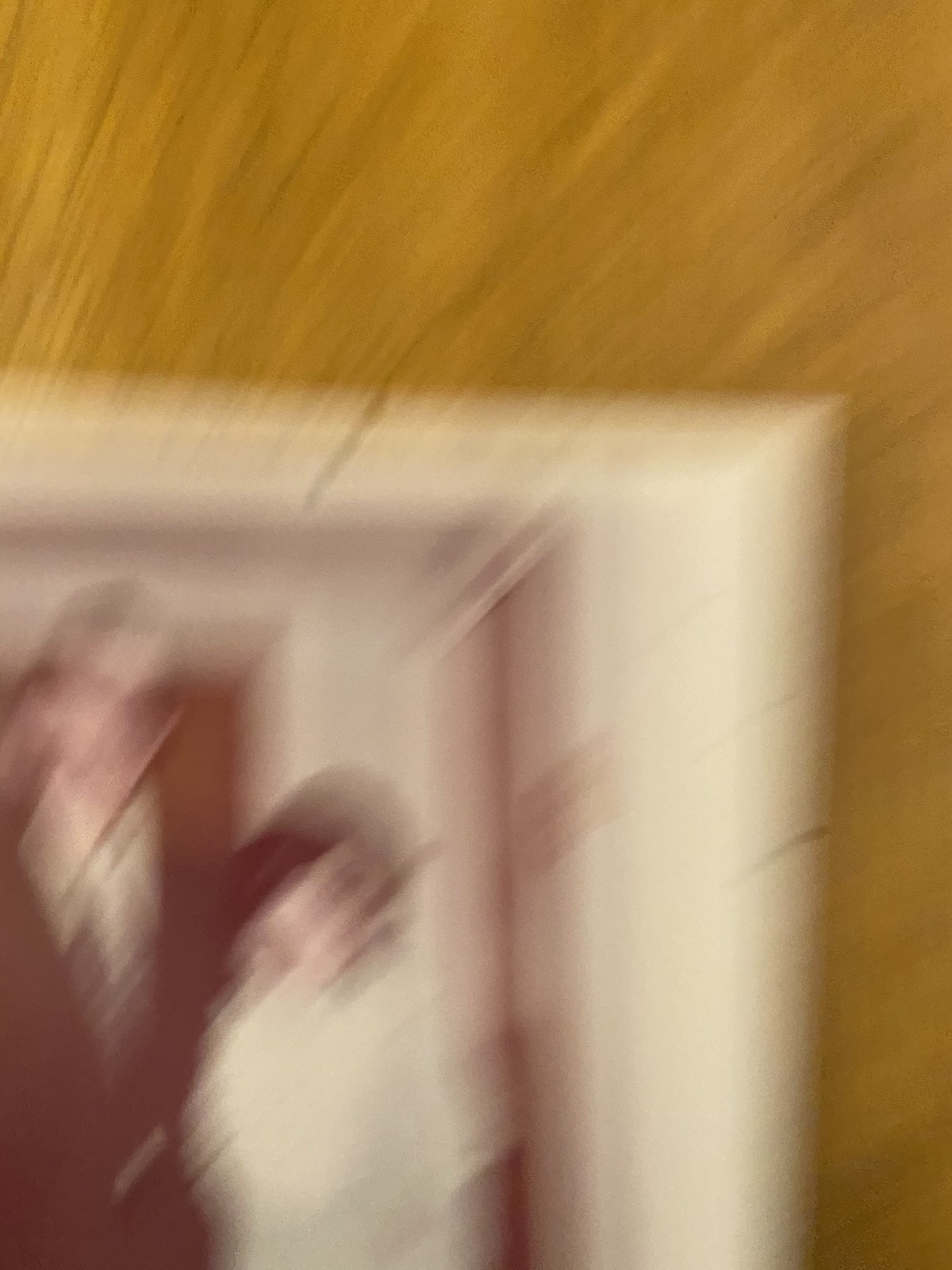This photograph, encased in a white frame and laying on a wooden surface, captures a low-quality, very blurry image of a man and woman standing in a doorway. The photo, which seems to be a vintage wedding or prom picture, reveals the couple from the waist up against a background of light tan walls. Both the doorway and door frame are white, contrasting with the brown wood paneled ceiling and walls surrounding it. The man, positioned on the left, appears much taller and is dressed in a suit with a white shirt and tie; he possibly has glasses and grayish hair. The petite woman on the right, with dark hair, is wearing a white outfit. Due to the severe blurriness and motion blur in the image, details of their faces and any background elements beyond the door are indiscernible.